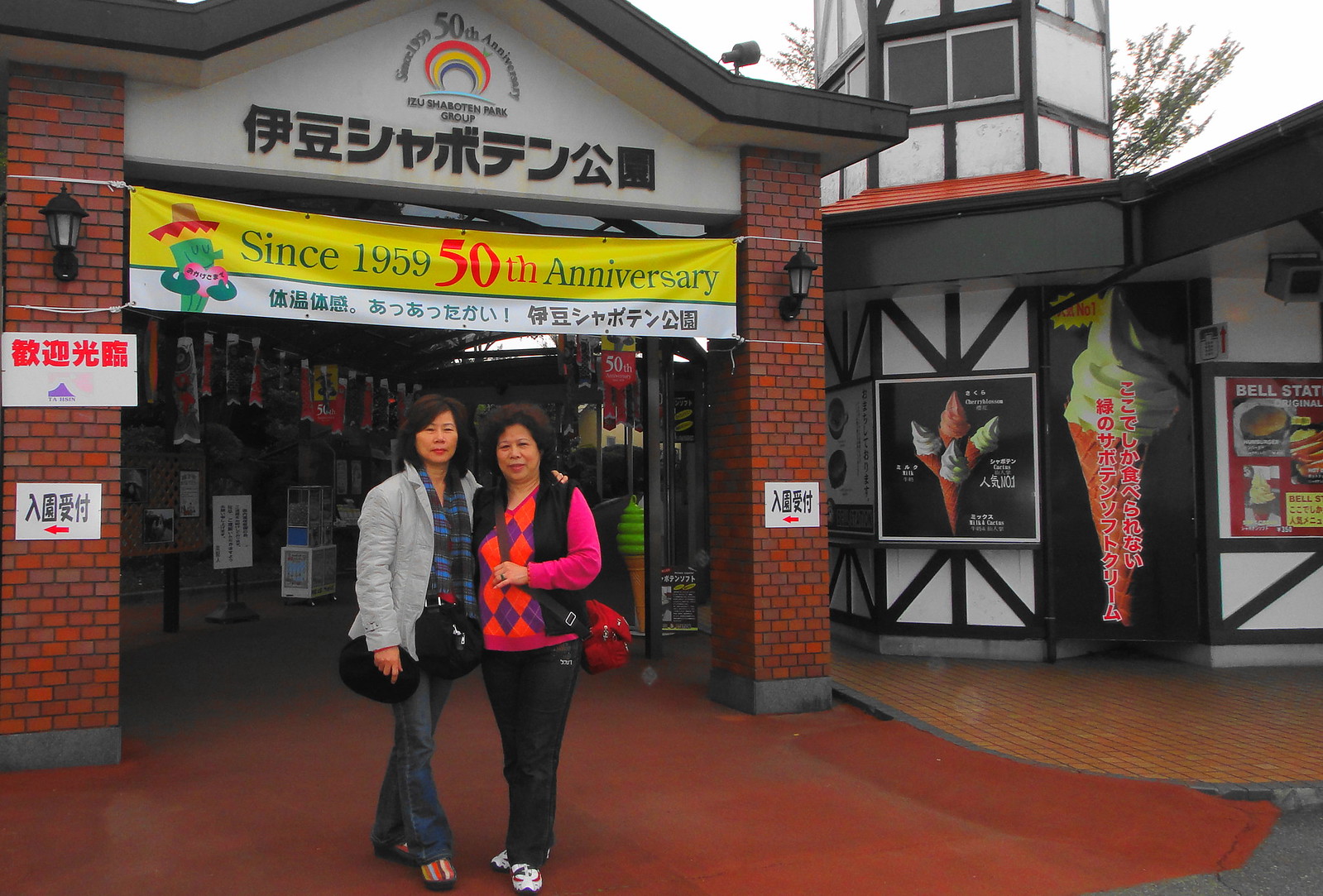Two middle-aged Asian women are standing in front of a vibrant storefront, possibly a supermarket or a venue. The storefront features numerous posters, many in Chinese or Japanese, and has bright colors that catch the eye. The building itself is painted white with black frames and has bricked pillars framing the entrance.

The woman on the left has shoulder-length hair and is dressed in a bright gray fall jacket over a blue and black striped sweater. She accessorizes with a matching blue and black scarf, blue jeans, and multicolored striped shoes. In her hand, she holds a black cap, and a black bag is slung across her front.

The woman on the right sports frizzy, curly hair. She wears a black vest over a pink sweater patterned with purple and red diamonds. She pairs this with black joggers and white trainers. She also has a bag slung across her chest. Both women are posing amicably, standing arm in arm.

The storefront sign prominently reads, "Since 1959, 50th Anniversary, Izu Shiboten Park Group," with Japanese characters below and a yellow banner featuring a cartoon cactus. An ice cream stand is visible to the right side of the entrance.